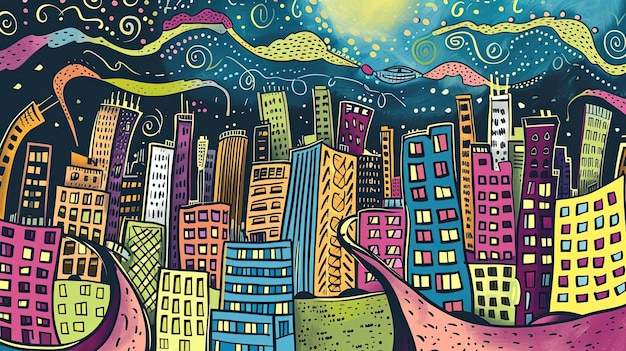This illustration presents a whimsical and stylized city skyline, with curvy and wobbly skyscrapers rendered in a vibrant palette including blue, red, yellow, orange, purple, pink, gray, and white. Emphasizing the playful, almost surreal nature of the scene, the buildings lack straight edges, contributing to a cartoonish, almost dreamlike quality. The dark blue sky above is reminiscent of Van Gogh's "Starry Night," filled with swirling lines that could be clouds or smoke, adding to the sense of movement. At the top of the image, a radiant yellow orb—possibly the sun or the moon—casts its light, creating an ambiguous, ethereal atmosphere. Accompanying the celestial body, colorful streamers and confetti fill the sky, enhancing the overall festive and surreal ambiance.